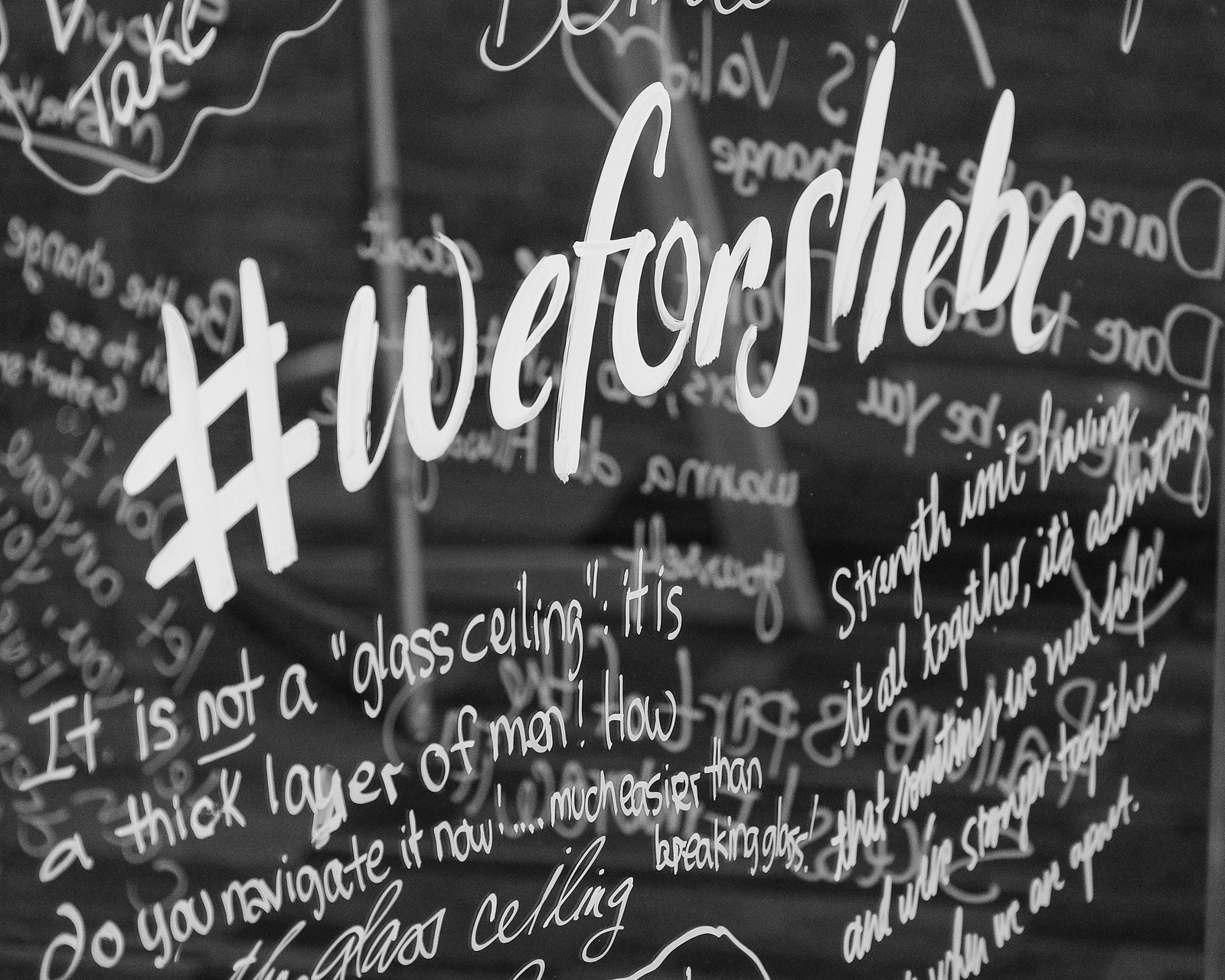The black-and-white photograph captures a pane of glass densely covered with handwritten, white-inked quotes and messages. The central feature is a hashtag, "#WeForSheBC," prominently written at the top. Various empowering statements are scattered across the glass. Notable quotes include, "It is not a glass ceiling. It is a thick layer of men. How do you navigate it now? Much easier than breaking glass," and, "Strength isn't having it all together. It's admitting that sometimes we need help and we're stronger together than when we are apart." The layered text, some visible on the opposite side of the glass, creates a sense of depth and complexity, reinforcing themes of solidarity and empowerment. The image, likely taken indoors or possibly at a business or residence, evokes a feeling of community and collective strength.